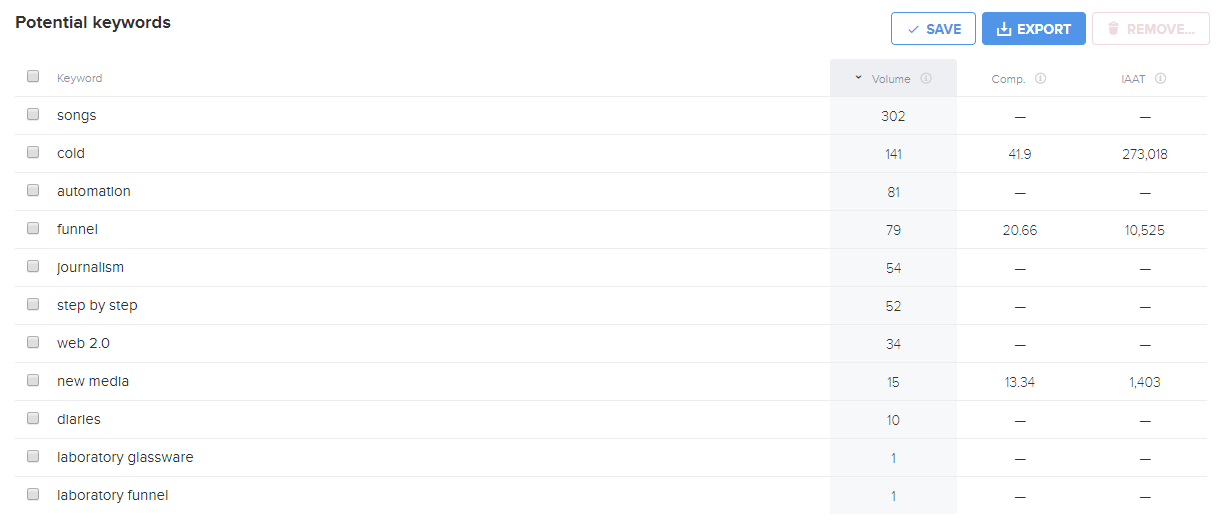Sure! Here’s a cleaned-up and detailed caption for the image described:

---

Screenshot of a detailed chart titled "Keywords Analysis." The chart features a series of essential keywords listed in a table format. Each keyword has an associated check box, although none of these are checked. The keywords listed include: songs, code, automation, funnel, journalism, step-by-step, web 2.0, new media, diaries, laboratory glassware, and laboratory funnel. 

For the keyword "songs," under the "Volume" column, there is a notation "volume comp in IAAT," with "302 comp" and dashes under the "IAAT" column. 

For the keyword "code," the volume readings are "141" under one column, "41.9" under another, and "273.018" in the last column. 

The keyword "automation" is associated with "81" in one column, with the remaining columns containing dashes.

For "funnel," the values shown are "79," "20.66," and "10.525" across the columns.

The keyword "journalism" has "54" in one volume column and dashes in the others, while "step-by-step" shows "52" with remaining values as dashes.

Additionally, the interface presents options including "Save" on a blue button within a white rectangle, "Export" on a blue and white button within a blue rectangle, and "Remove" on a button within a white rectangle. The interface also uses a faint red color to highlight some elements.

---

This caption provides a comprehensive and clear description of the chart and its elements.